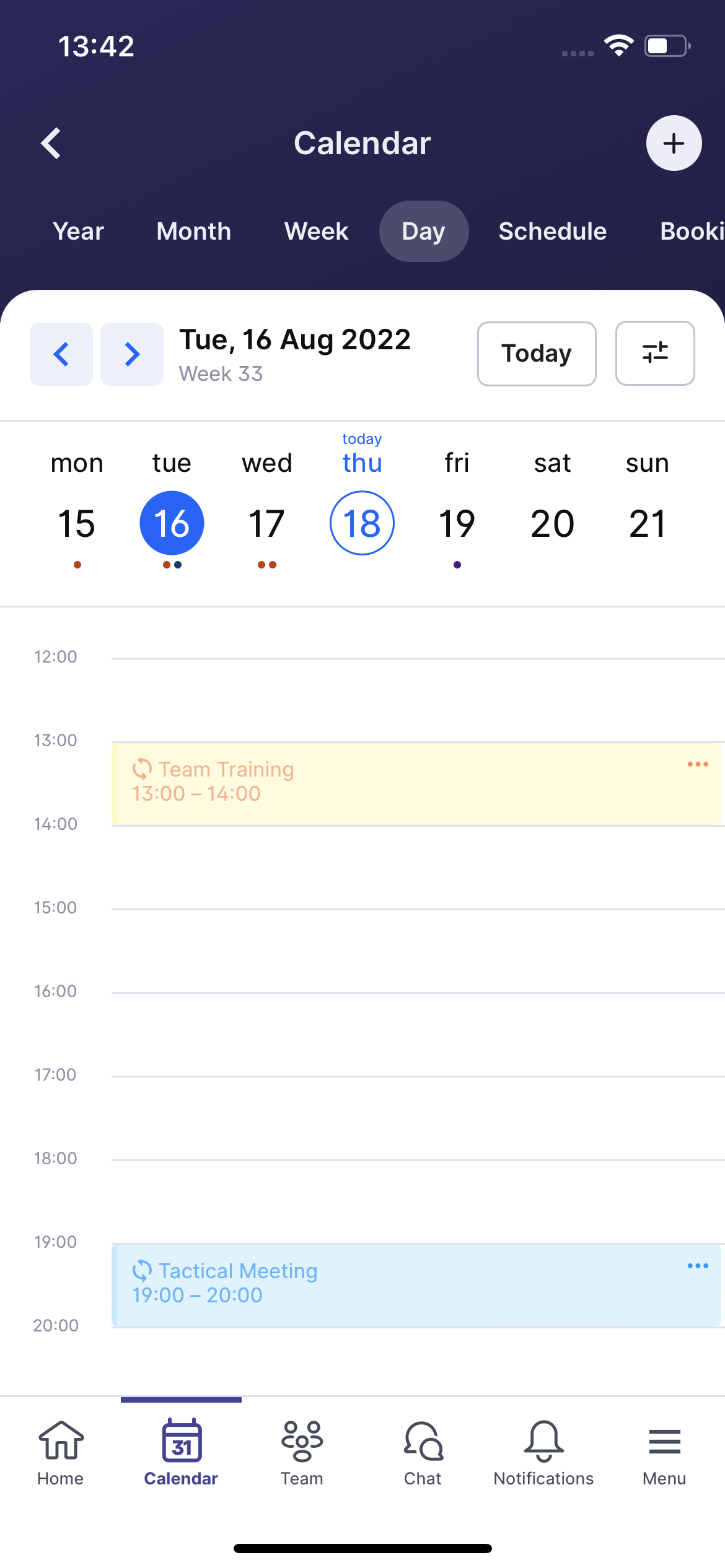The image depicts a smartphone screen showcasing a calendar app with a dark blue header where the word "Calendar" is prominently displayed in white text. The top section of the app features navigation options listed horizontally in white text, starting with Year, Month, Week, Day, Schedule, and Booking from left to right. On the top right corner, there's a circular white button with a plus sign, allowing users to add events, while the top left corner features a back arrow for navigation.

Beneath the header, the main calendar interface is set against a white background with black text. The current date area indicates "Tuesday, 16 August 2022, Week 33," with the days of the week listed from Monday to Sunday, spanning dates from the 15th to the 21st of August. The date "Tuesday" is highlighted in blue, indicating the current day. The Thursday date (18 August) is circled in blue, emphasizing an important event.

A scheduled event on Thursday is detailed beneath the date: a team training session from 1 PM to 2 PM, highlighted with yellow and orange for emphasis. Additionally, a technical meeting is scheduled from 7 PM to 8 PM, detailed in blue text. 

At the bottom of the screen are navigation tabs or buttons, including Home, Calendar, Team, Chat, Notification, and Menu. Only the Calendar tab is highlighted in dark blue, indicating the current view, while the others remain unhighlighted in grey.